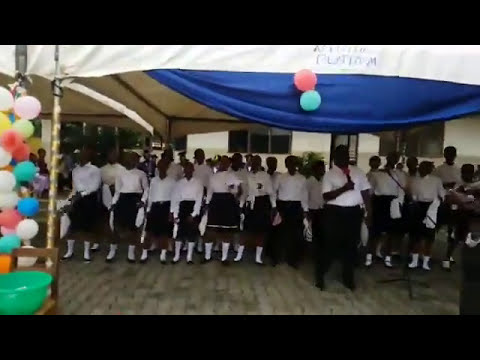In the image, a group of African American individuals, dressed uniformly in white long-sleeved tops paired with either black pants or skirts and white socks, are gathered under a blue-roofed tent. The scene hints at a celebration or event, with colorful decorations such as aqua, pink, yellow, blue, and green balloons adorning the left side. The backdrop features a white building with windows, suggesting an outdoor setting, possibly near a school. Prominently in the foreground is a man holding a microphone, also dressed in the same white and black attire, appearing to address the group. Elements such as a green plastic bowl, a silver pole, and a wooden chair are situated nearby. The tent’s covering creates a blue canopy over the group, and the floor beneath them is made of wooden panels. The main colors in the image are black, white, blue, with accents of green, pink, yellow, and a hint of orange, all framed by black bars at the top and bottom of the picture.